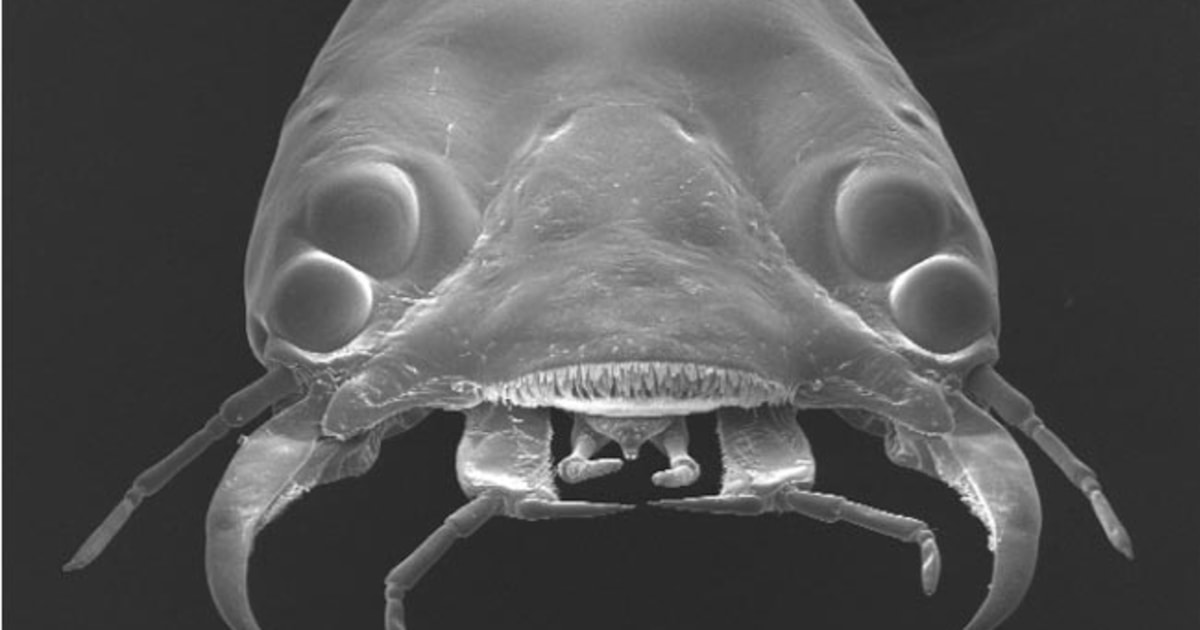The image depicts a detailed, close-up view of a crab-like crustacean, captured in shades of white, black, and gray, suggestive of an x-ray or night vision photograph. The creature, exhibiting a textured surface, faces the camera against a solid black background, emphasizing its translucent yet detailed features. It possesses two large pincer claws located beneath its four eyes, and several other appendages: two long legs extending from either side of its eyes, and multiple smaller pincer claws and legs, summing up to around eight visible limbs. The frontal region is bulbous, with a large mouth obscured by what appears to be hair, giving the impression of an opening lined with teeth. Overall, the creature's ghostly appearance, combined with its distinctive anatomical details, evokes the eerie image of a sea creature caught mid-motion.